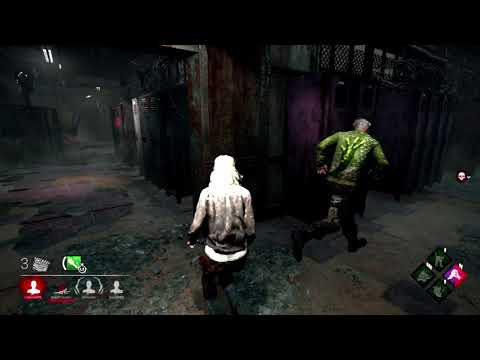The image is a dark, disturbing screenshot from a horror video game, possibly on a PC. It features two characters in a grim setting with dirty, disgusting floors and purple metal lockers. One character, centered at the bottom with long white hair, appears to be running to the left. The character on the right side is dressed in a green jacket, black pants, and boots, and might be running away. The scene evokes a sense of mystery and horror, akin to games like Resident Evil or The Evil Within. Bathroom stalls and lockers characterize the room, adding to the unsettling atmosphere. The bottom left corner of the screen displays an interface with a red-lit icon and a green-lit icon, potentially indicating player status or items available for use. The screen is framed with black rectangles at the top and bottom, enhancing the cinematic quality of the game.